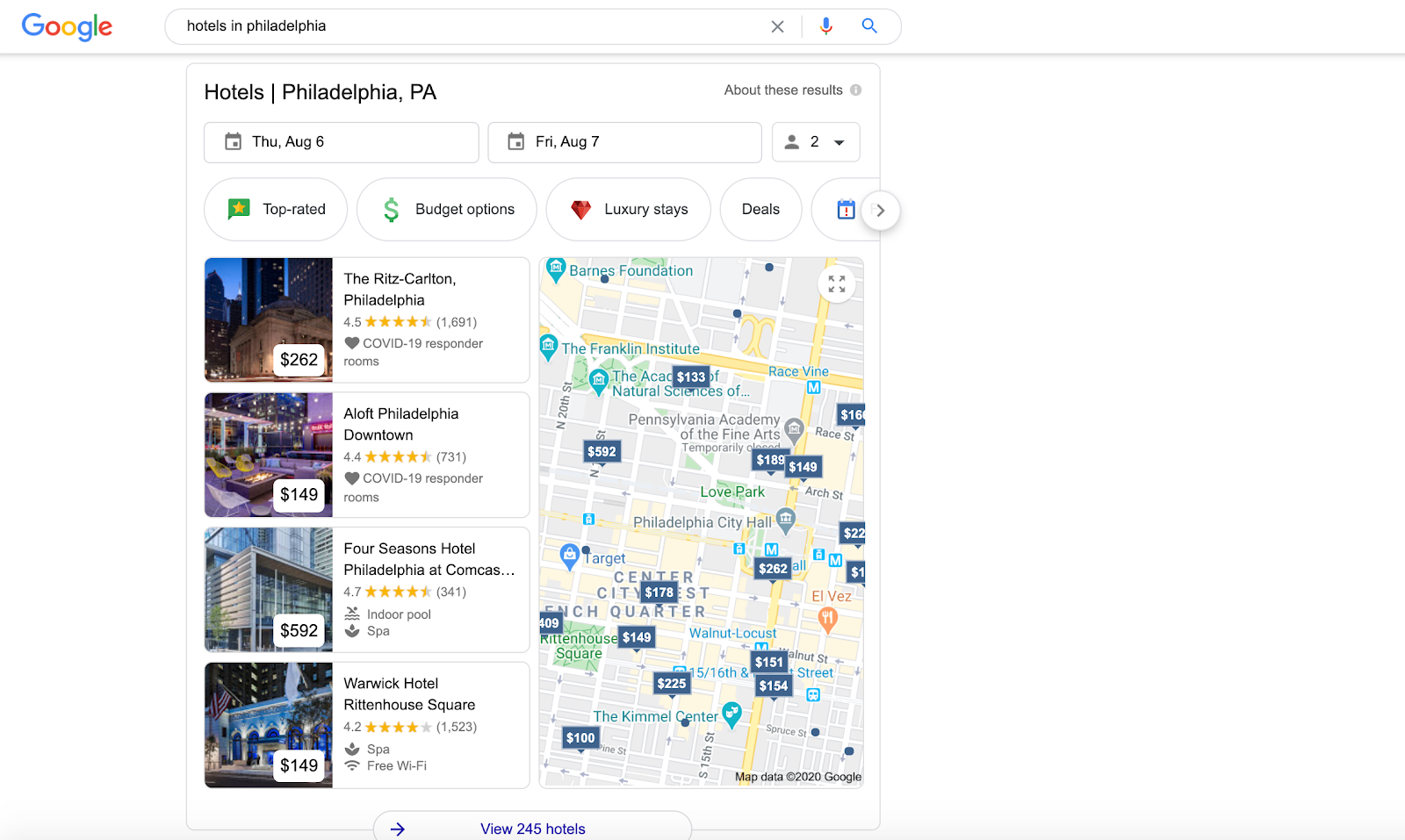The image depicts a Google search results page for "hotels in Philadelphia". The layout is characterized by substantial empty space, contributing to its large appearance. The top of the page features a distinct oval search bar with the query "hotels in Philadelphia" prominently displayed in black text towards the left.

Just beneath the search bar, there is a small rectangular section that presents the actual search results. In the top left corner of this section, the text "hotels in" is rendered in a basic sans-serif black font, followed by a line divider. Below this, the text "Philadelphia, PA" appears, with both "Philadelphia" and "PA" capitalized.

The search results section is divided into two equally-sized rectangular areas, outlined in light gray. The left rectangle contains a calendar with the date "THU, AUG 6", whereas the right rectangle displays "FRI, AUG 7". To the right of these date selectors, there is a smaller rectangular area, also outlined in light gray, featuring a gray silhouette icon of a user and the number "2". A black downward-pointing arrowhead indicates that this menu allows the selection of a different number of guests.

Below these rectangular selections are several filter options, each displayed in oval shapes with white backgrounds and light gray borders. The filter options include "top-rated", "budget options", "luxury stays", and "deals". There is another oval-shaped icon featuring a blue calendar with an orange exclamation point, but its label is partially cut off and unreadable.

Following the filter options, the image lists various hotels in Philadelphia. The first listed hotel is "The Ritz Carlton, Philadelphia", followed by "Aloft Philadelphia Downtown", "Four Seasons Hotel Philadelphia", and "Warwick Hotel Rittenhouse Square".